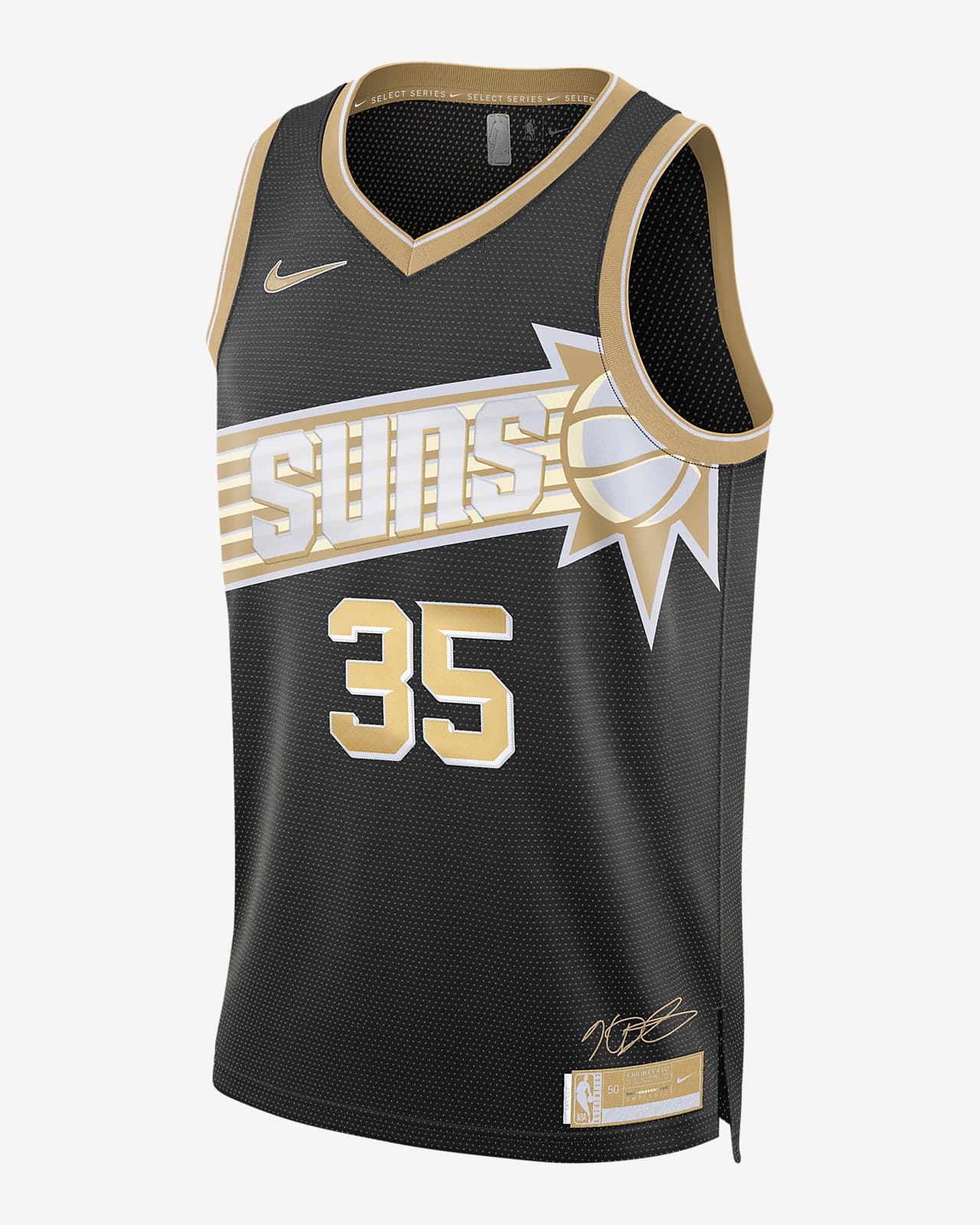This image showcases a black sleeveless basketball jersey against a plain white background. The jersey, designed by Nike, features distinctive tan and white trim around the collar and armholes. Prominently displayed on the front is the word "Suns" in white text, set against a horizontal tan and gold band. Beside the "Suns" logo is a dynamic graphic of a white basketball, accented with golden jagged rays, giving the impression of the ball in motion. Below the logo is the number 35, presented in gold with a white outline and a shadow effect. At the very bottom of the jersey, a player's signature, seemingly "KDB", is visible, along with a gold label on the bottom right that includes the NBA logo and a gold check mark. The jersey appears to be an item for sale, as indicated by the professional, isolated presentation of the photograph.